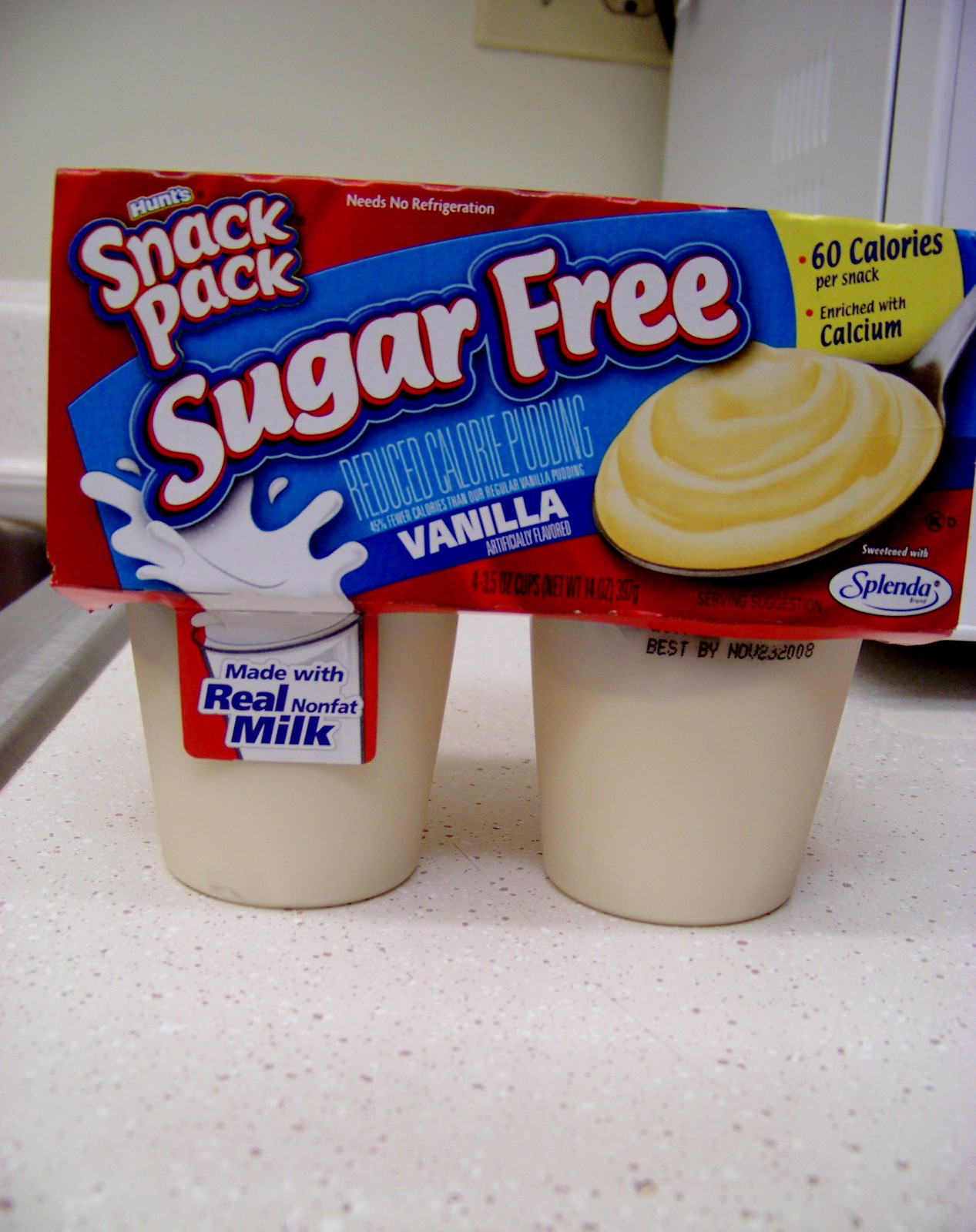A photograph taken in a kitchen shows a package of Hunt's Snack Pack sugar-free vanilla pudding prominently positioned at the center. The packaging, which can hold four cups, is distinctive with a predominantly red design featuring a blue rectangle running across the top. In large white text with red and blue outlines, it declares the pudding as sugar-free, made with real nonfat milk, and sweetened with Splenda. The front of the pack also emphasizes that each snack contains just 60 calories and is enriched with calcium. You can see a spoon with creamy vanilla pudding depicted on the packaging. Additional text on the package informs that it requires no refrigeration. The package sits on a kitchen counter with a beige-ish, speckled pattern, and the background includes glimpses of a fridge and a stove, partially cut off by the image frame.